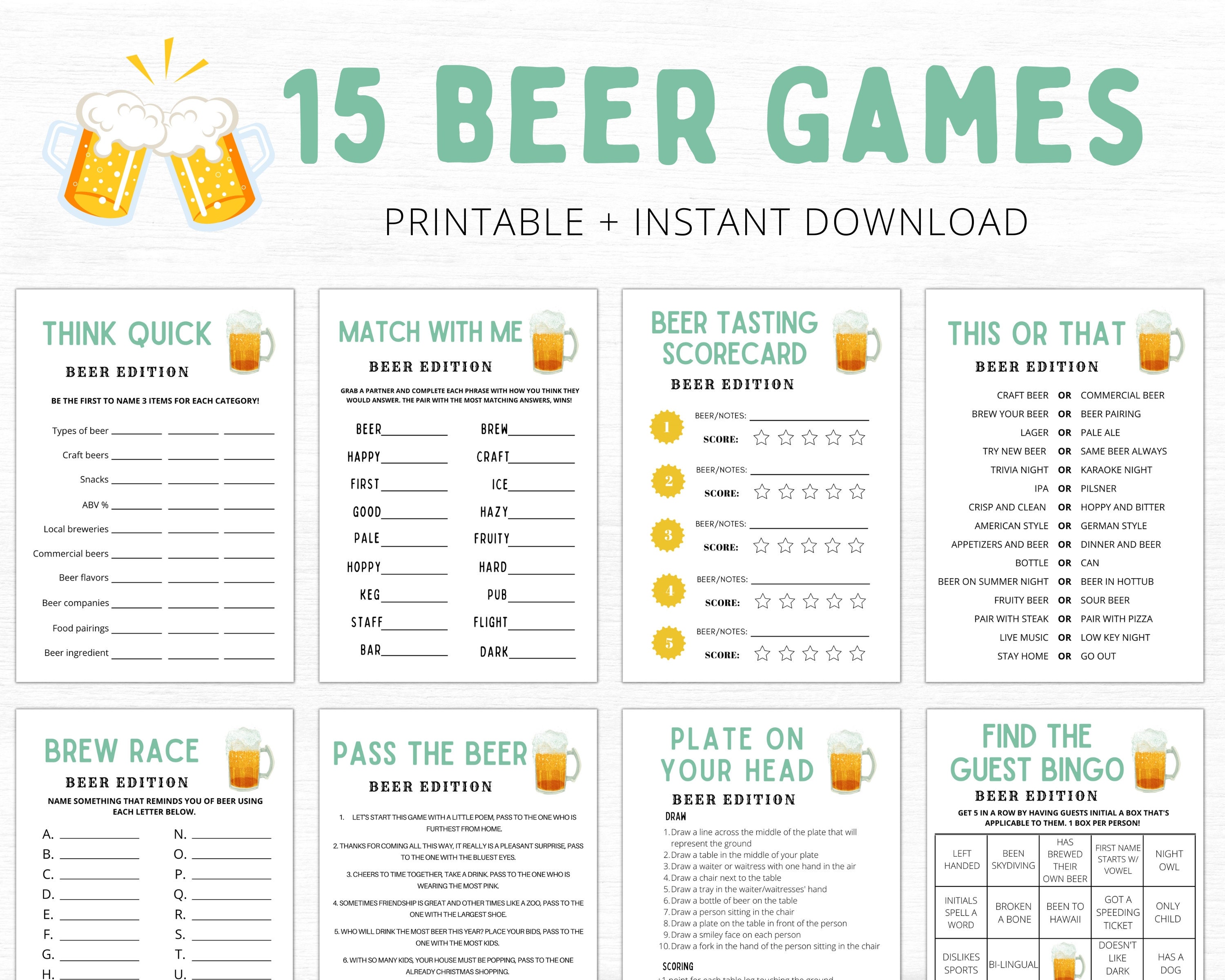This image showcases a printable and instant-download chart featuring 15 different beer-themed games. At the top, "15 Beer Games" is prominently displayed in light green text against a white background. Beneath this, smaller black text reads "Printable" and "Instant Download." In the upper left corner, there is a cartoon image of two foaming beer steins clinking together. The chart is organized into two rows of four game cards, although the bottom row is partially cut off in the image.

The top row of game cards includes:
1. **Think Quick, Beer Edition** - A game detailing various beer types.
2. **Match With Me, Beer Edition**.
3. **Beer Tasting Scorecard**.
4. **This or That**.

The bottom row features:
1. **Brew Race**.
2. **Pass the Brew**.
3. **Play It on Your Head, Beer Edition**.
4. **Find the Guest Bingo** - Featuring various attributes where participants may write specific details.

These printable game cards generally have white backgrounds with black text, some featuring blank spaces to fill in details, and are visually organized for easy reading and use during beer-themed events.